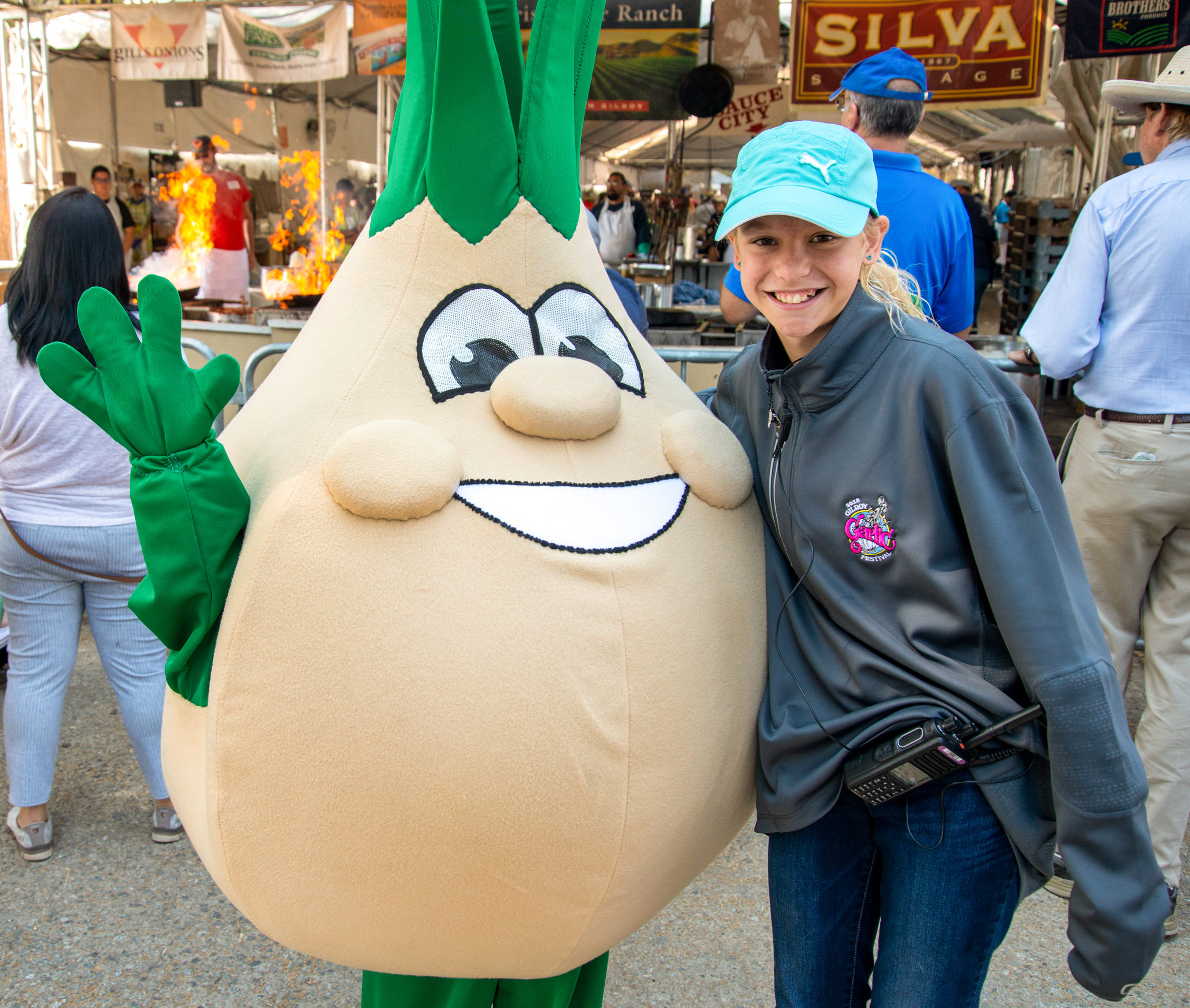In this vibrant photo taken at what appears to be an agricultural fair, a young girl, likely around 10 to 12 years old, is warmly posing with a character dressed as a garlic or onion. The mascot, characterized by its large, white and green face with expressive big eyes, green legs, hands, and "hair," brings a whimsical touch to the event. The girl, smiling brightly despite her slightly crooked teeth, wears a light blue Puma baseball cap adorned with the brand's white cat logo. Her wavy, blonde hair is neatly pulled back, and she accessorizes with small blue earrings. Bundled in a gray zip-up sweatshirt that's a bit oversized for her small frame, she also sports well-worn denim pants with a walkie-talkie clipped to her left hip. In the backdrop, a bustling scene unfolds with several tents, possibly indicating cooking demonstrations, as evidenced by visible flames and observers gathered behind a barrier. The lively atmosphere adds a dynamic context to this joyful moment captured amid the fair's festivities.